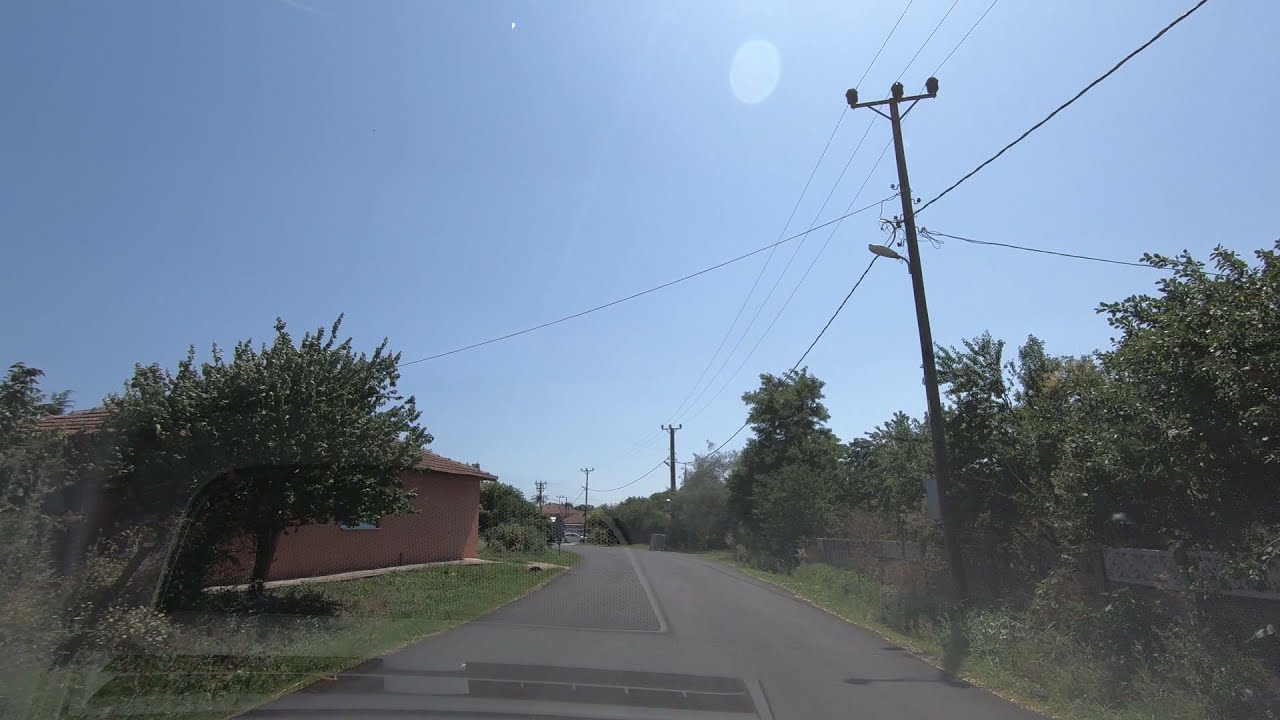The image captures an outdoor scene during daytime, likely taken from a dash cam within a moving vehicle on an empty road. The sky is a clear, vivid blue, and green trees line both sides of the road. On the left side, nestled among the trees, partially obscured by foliage, is a house painted in shades of red or orange. Utility poles stand along the right side of the road, and in the far distance, another house can be seen at the horizon where the road continues. The overall image boasts a high level of clarity and rich colors, with no visible people, numbers, or letters, and is well-lit by natural daylight.